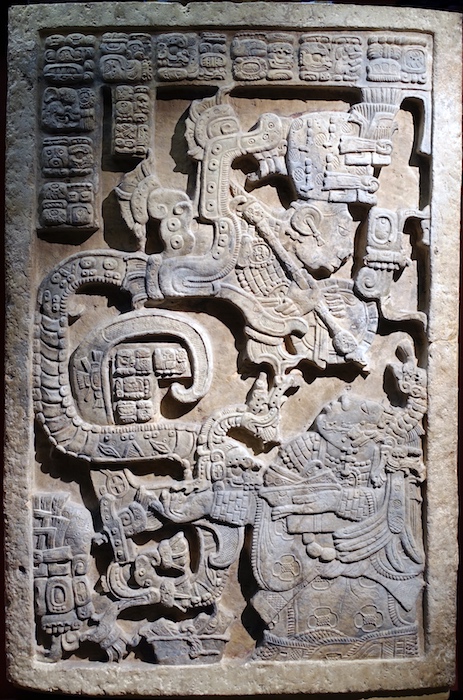The photograph captures a detailed stone carving, likely of ancient origin. The rectangular stone, predominantly gray with light brown hues, is meticulously engraved, showcasing a mythological scene. At the top of the carving, a stylized dragon, possibly symbolizing a deity or mythical creature, dominates the artwork. The dragon's tail gracefully winds around the lower portion of the stone. Below the dragon, a man with an elongated, serpent-like waist holds a staff, his regal appearance emphasized by a crown and ornate clothing. Another man stands gazing up at this serpent-man figure. Surrounding the main figures, the stone features intricate designs, including representations of baskets, musical instruments, regalia, weapons, and various other day-to-day objects. The upper left corner is adorned with hieroglyphic-like symbols and stylized images of small animals and humanoid faces, arranged in pairs and spread across the top. The entire scene is bordered by a solid stone frame, enhancing the intricate artistry of the ancient carving.